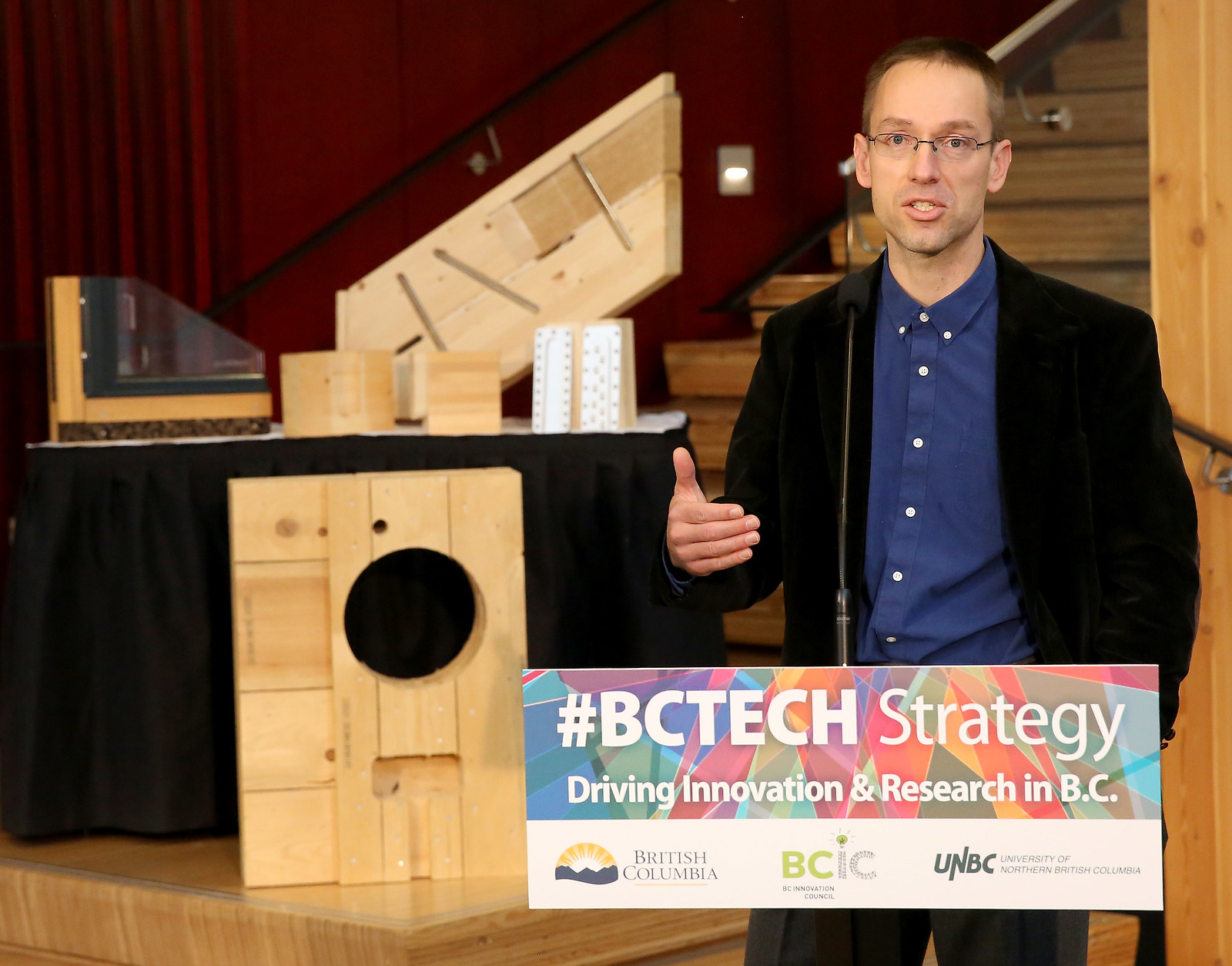The image captures a Caucasian man giving a speech, facing the camera with his mouth open mid-speech. He is positioned on the right side of the frame, gesturing expressively with his right arm extended while his left arm hangs down. The man sports brown hair, glasses, a black jacket, a button-down blue shirt, dark pants, and is light-skinned. He stands in front of wooden stairs and next to a table that features an intricate wooden model, including a rectangular piece with a circular hole. Behind him, there's a bold red wall and various colorful geometrical shapes forming a rainbow pattern with colors such as red, yellow, green, purple, blue, and brown. Notably, a text banner at his waist reads, "#BC Tech Strategy, driving innovation and research in BC," accompanied by logos for BCIC, UNBC, and a sunrise motif representing British Columbia.